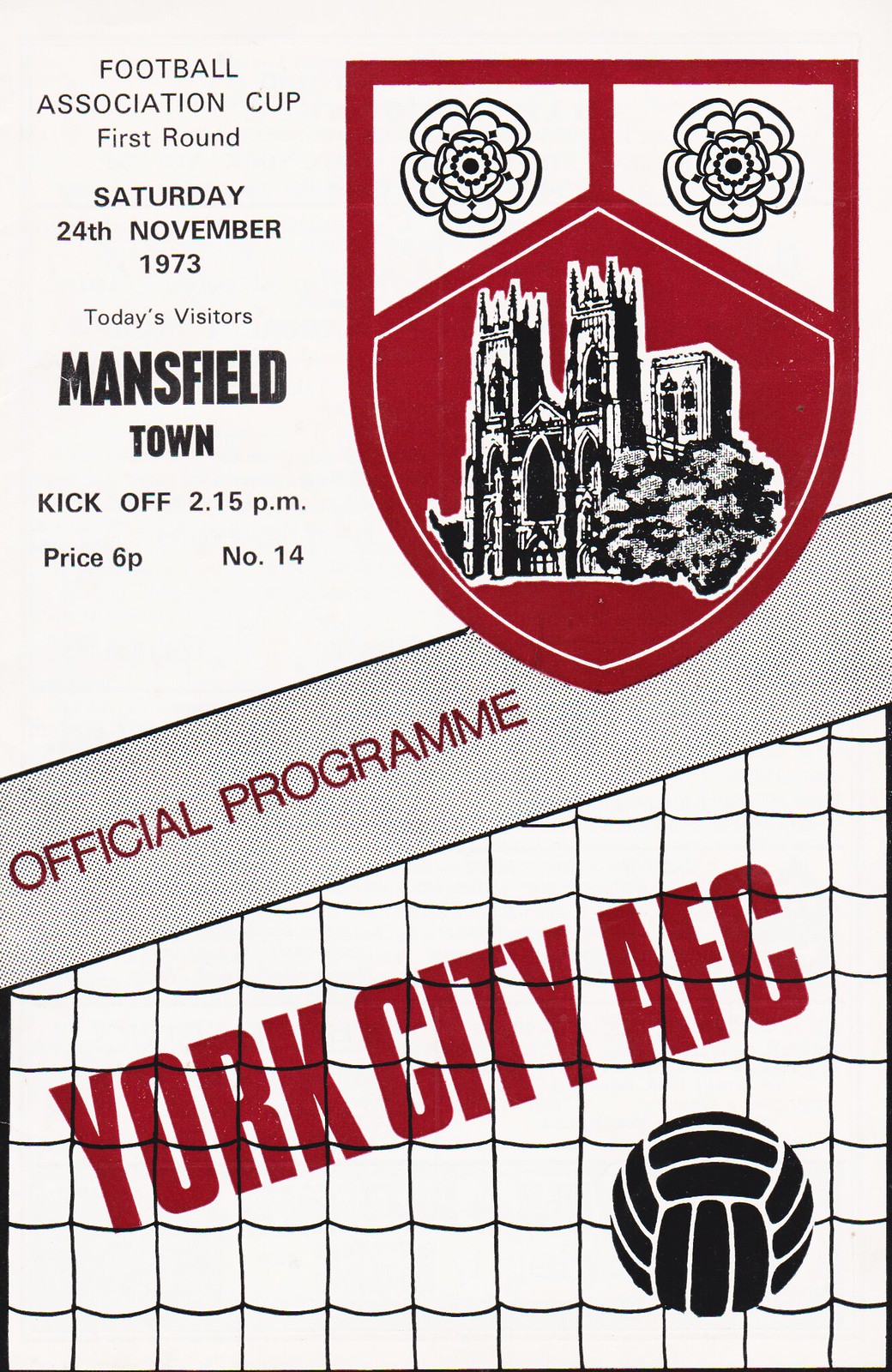The image appears to be the cover of a vintage football match poster or magazine. In the top right corner, there's a detailed crest—a shield featuring two white flowers at the top, and below them, a black illustration of a church or castle with two towers set against a red background. To the left of the crest, the text reads "Football Association Cup first round, Saturday 24th November 1973,” followed by “Today's visitors Mansfield Town, kickoff 2.15 p.m., price 6p, number 14.” A gray banner with black edges spans diagonally across the middle, inscribed with "official program" in a red or burgundy font. Beneath this banner, there’s an image of a soccer net with a soccer ball icon, accompanied by the prominent text "York City AFC."